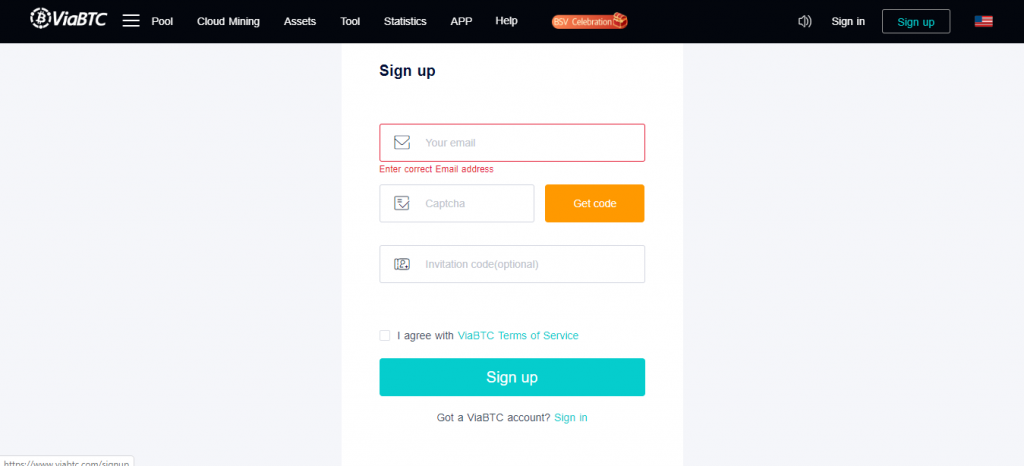The screenshot displays the homepage of a website named "ViaBTC." In the upper left corner, the ViaBTC logo—a small circle—accompanies the site name. A horizontal black banner at the top hosts the main navigation menu items: Pool, Cloud Mining, Assets, Tool, Statistics, APP, and Help. To the right of these options, there's an orange button labeled "Calculation," followed by a speaker icon, and the options to Sign In or Sign Up. An American flag icon indicates that the language setting is currently English.

The "Sign Up" option is highlighted in blue, suggesting it is currently selected. Below the banner, the central part of the screen features a grey background with a prominent white sign-up dialog box. This box has a red rectangle around the email address input field, emphasizing where users need to enter their email to proceed with registration. There is also an orange button labeled "Get Code" for CAPTCHA verification. Beneath this, users can input an invitation code, if they have one, followed by a checkbox for agreeing to the site's terms and conditions. Completing the registration process involves clicking a blue "Sign Up" button at the bottom of this dialog box.